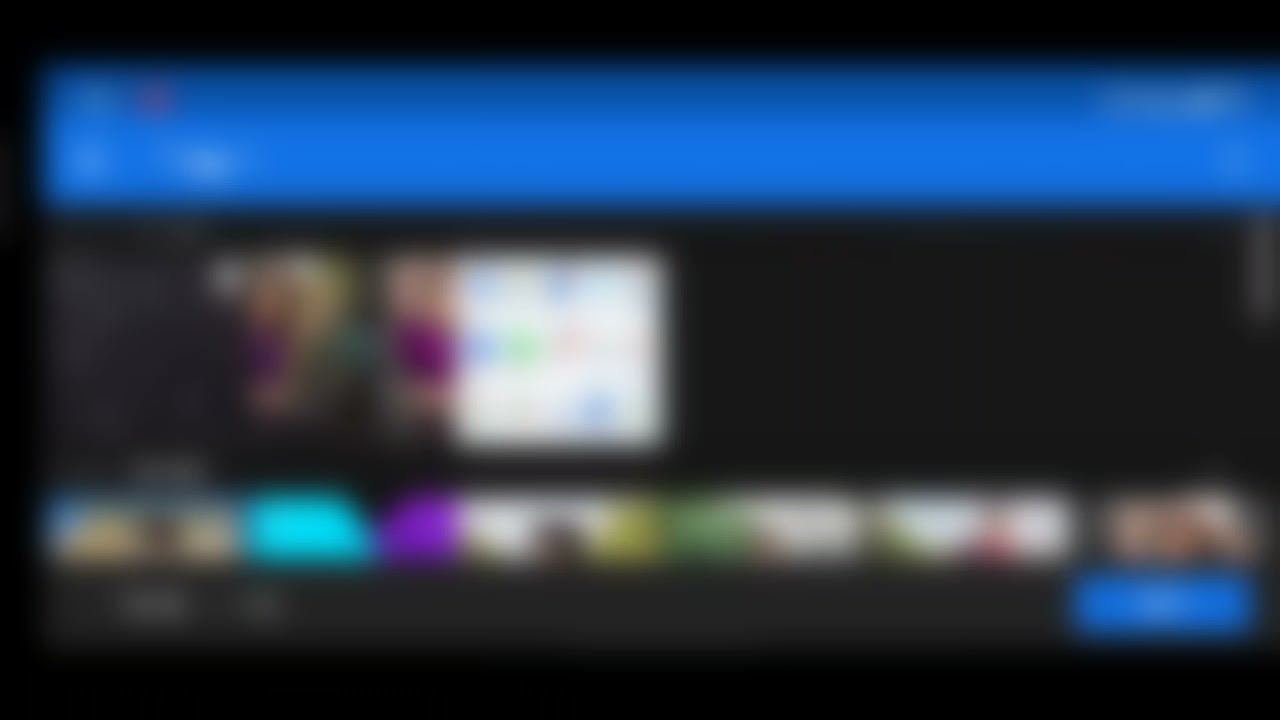This image, though very blurry and thus hard to make out, appears to show an interface possibly from a streaming service menu on a computer, tablet, or smart TV. The screen is framed by a black border at the top and bottom, with a noticeable blue bar across the top. In the central part of the image, there seems to be a larger highlight or preview window, likely displaying a selection from the menu. The preview includes an image featuring two girls, one of whom seems to be wearing a pink or purple shirt and may have blonde hair. There are thumbnails or smaller images along the bottom of the screen, presumably showcasing different shows or movies available for selection. The bottom right corner shows what appears to be a blue button, likely serving as an "OK" or selection button, accompanied by navigational arrows to its left for scrolling through options. Overall, despite the blur, we can discern a typical streaming service interface with various selectable content.